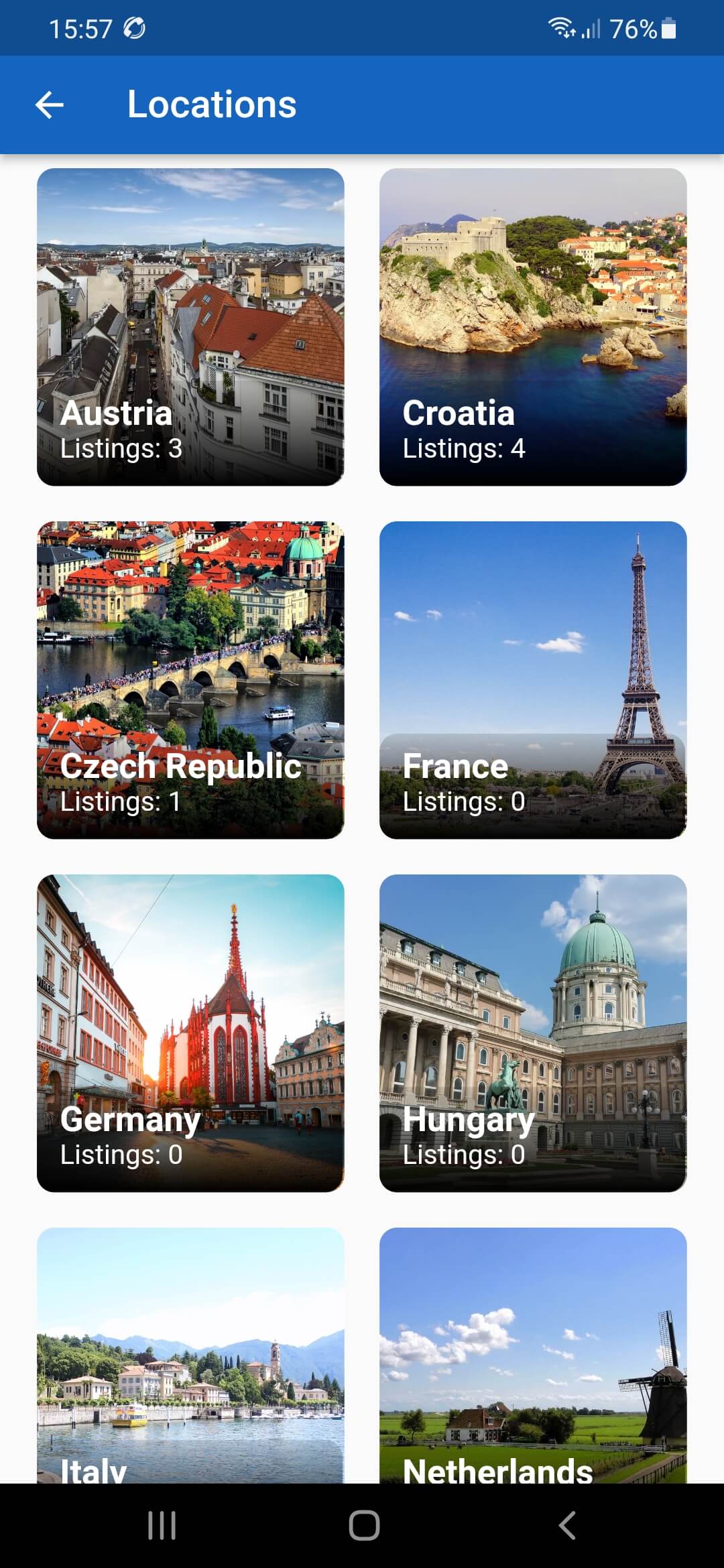This image is a screenshot taken from a cell phone. At the top of the image, there is a dark navy rectangular strip that spans the width of the screen. Just below it, there's a lighter, royal blue rectangle. In the royal blue section, there's text that reads "Locations," accompanied by a left-pointing arrow.

Below these strips, the main content area displays eight photos, each representing different countries and their notable locations, along with the number of active listings for each:

1. Austria: The photo indicates there are 3 listings.
2. Croatia: The image showcases a beautiful landscape with water features, indicating 4 listings.
3. Czech Republic: This section indicates there is 1 listing.
4. France: Featuring an image of the Eiffel Tower, this section indicates there are no active listings.
5. Germany: This section also shows 0 listings.
6. Hungary: Similarly, Hungary has 0 listings.
7. Italy: The listing count is not fully visible.
8. Netherlands: The listing count is also obscured by a black bar.

At the bottom of the screen, there's a black rectangular bar with various icons. In the center is a square icon, to the left are vertical lines, and in the bottom right corner, there's a left-pointing arrow icon. The lower part of the images for Italy and the Netherlands are partially obscured by this black bar, cutting off the listing information.